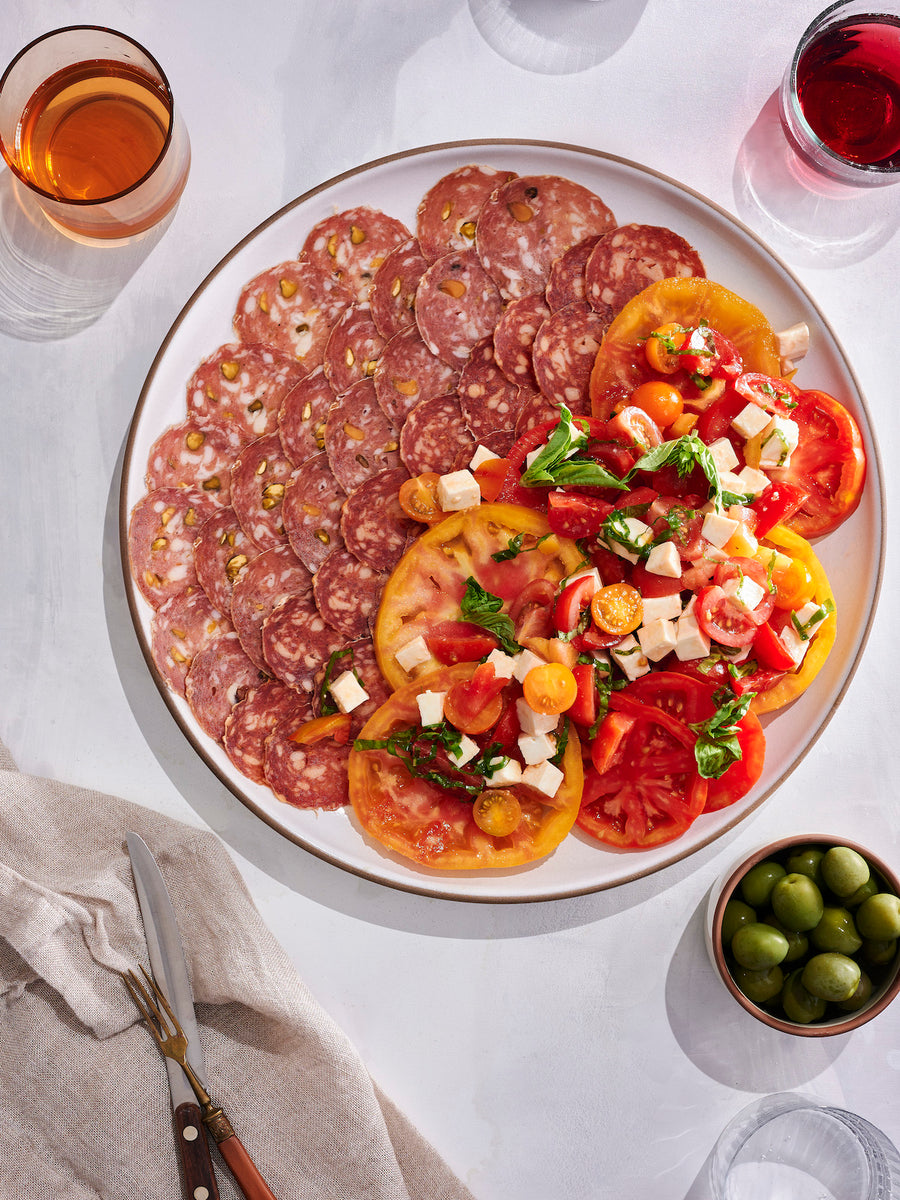In this overhead photograph, a white ceramic plate with a bronze rim rests at the center, showcasing a meticulous yet inviting charcuterie board arrangement. The left half of the plate features an assortment of salami or pepperoni slices, while the right half displays a vibrant mix of tomato slices, ranging from large yellow-red tomatoes to smaller cherry tomatoes, with cubes of feta cheese and scattered green herbs adding texture and flavor. To the top right and top left of the plate, two glasses of liquid are positioned, one filled with a rich red drink and the other with a golden amber beverage. Adjacent to the plate on the bottom right sits a small bowl brimming with green olives. To the left, a linen napkin accompanies dining utensils, including a sharp knife and a small, antique bronze fork, creating a balanced and picturesque setting on a white table.